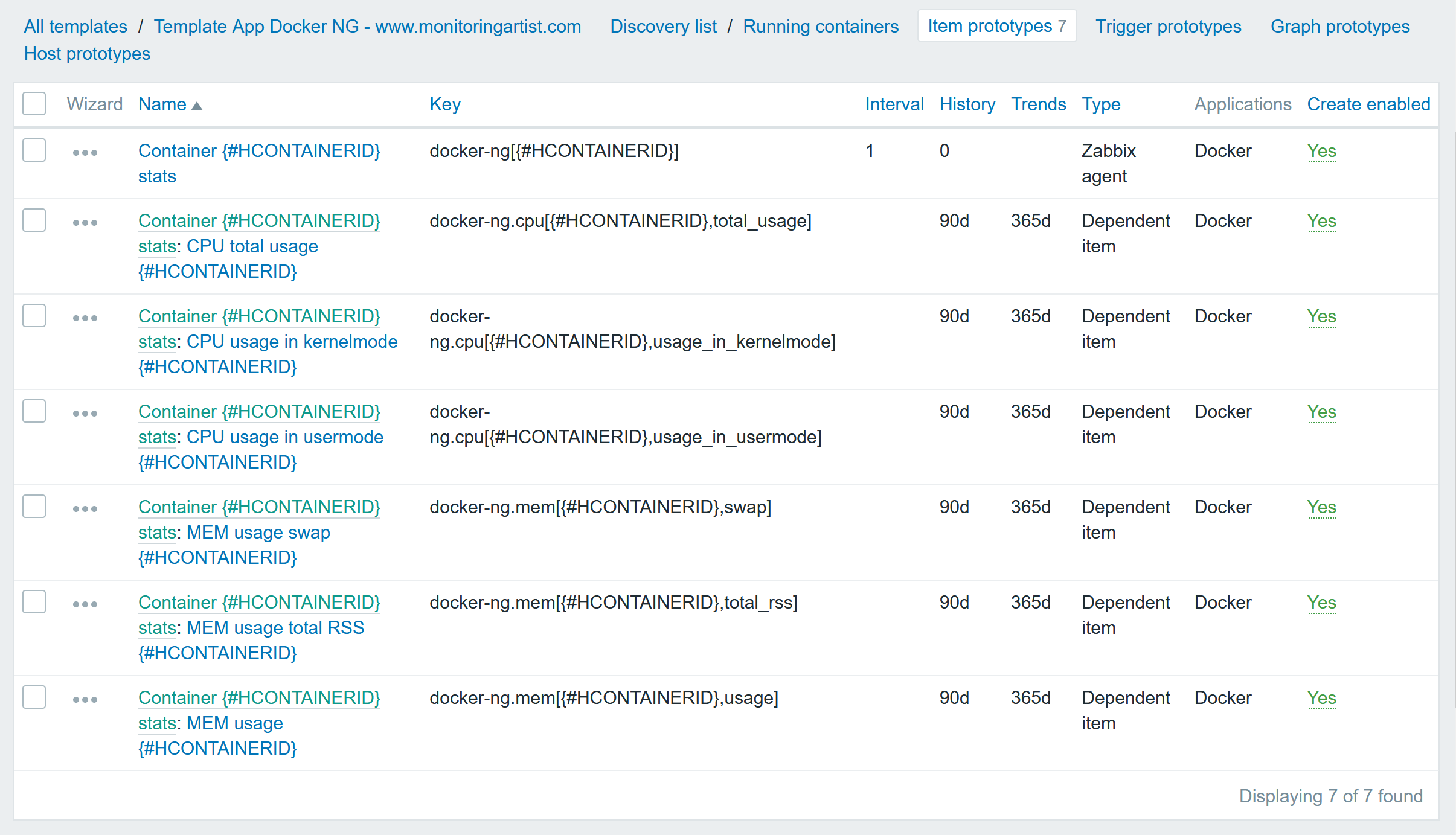The image features a detailed interface design against a white background. The layout displays item prototypes in blue, with seven items in gray. There is a row of checkboxes, and an interactive wizard symbolized by three vertical dots, as well as three horizontal dots. 

Key sections are labeled as Name, Key, Interval, History, Trends, Type, Applications, Create, and Enable. Each item’s processes are detailed in text form. The Create and Enable section consistently shows green check markers for 'yes,' while the Applications section indicates all items related to Docker.

### First Item Details:
- **Name**: `Container`
- **Key**: `#H-CONTAINER-ID` (all uppercase)
- **Stats**: Displayed for `docker-ng` with `[Container ID]` in brackets.
- **Intervals**: Set to 1
- **History**: Set to 0
- **Trends**: No data available
- **Type**: Zabbix Agent

### Second Item Details:
- **Name**: `Container`
- **Key**: `#H-Container-ID`
- **Stats**: CPU total usage, with `#H-Container-ID` in parentheses

Each section is meticulously itemized, ensuring clarity in monitoring Docker container statistics and corresponding Zabbix agent data.